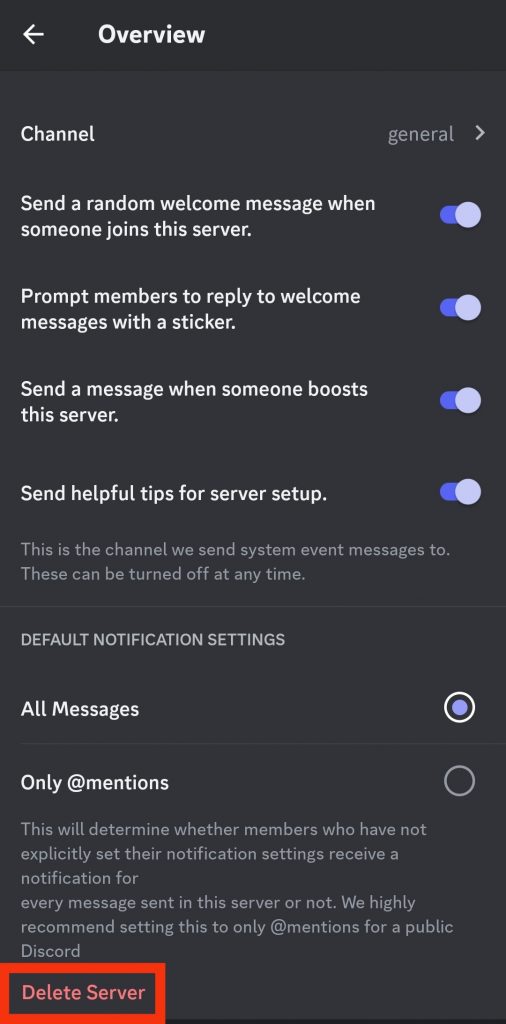This image is a vertical screenshot of a Discord interface in portrait mode. The top section has a dark black background featuring a white back button and the bold text "Overview." Below this section, extending downwards in a long column with a slightly lighter black background, is an organized list of settings.

At the top of this column, the section starts with the label "Channel" on the left and a forward arrow next to "General" on the right. This is followed by four rows of settings, each ending with a toggle button currently switched to "on," indicated by a blue color. The settings listed are:
1. "Send a random welcome message when someone joins the server."
2. "Prompt members to reply to welcome messages with a sticker."
3. "Send a message when someone boosts this server."
4. "Send helpful tips for server setup."

Subsequent to the toggles, in difficult-to-read gray text against the black background, a note reads: "This is the channel we send system event messages to. These can be turned off at any time."

Further down, there's a section titled "Default Notification Settings" with two options:
- "All Messages," which is checked on.
- "Only @mentions," which is not checked.

A brief explanation follows, stating that this setting determines if members who haven't set their notification preferences receive a notification for every message in the server. It suggests setting this to "Only @mentions" for public servers.

In the bottom left-hand corner, in red text, is an option to "Delete Server," highlighted prominently in red. Overall, the main focus of this screenshot is on how to manage and delete a server within Discord.